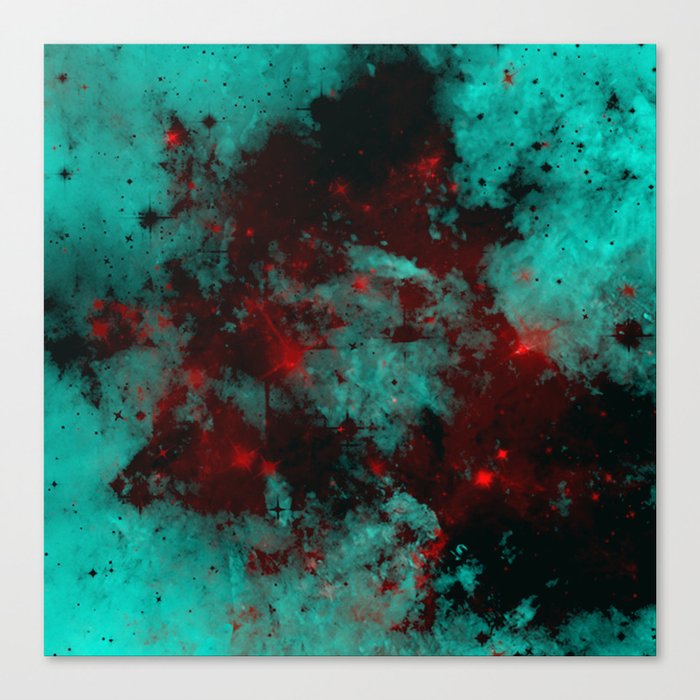The image features a vibrant and detailed abstract painting on a teal background. The composition is dominated by dynamic splatters and splotches of red and black paint. The black elements appear to have a smoky texture, with some areas showing more spread and blending, while others consist of individual spots. The red splatters resemble explosive bursts, as if shot from a paintball gun, adding a dramatic contrast to the teal. Scattered amid the vibrant colors are small, shiny red and black jewel-like elements, enhancing the complexity of the piece. Overall, the image, set against a slightly larger white square canvas, is clear and brightly lit, allowing the intricate interplay of colors and textures to stand out. This abstract painting, devoid of any text or signatures, makes for an eye-catching and thought-provoking artwork suitable for display on a wall.